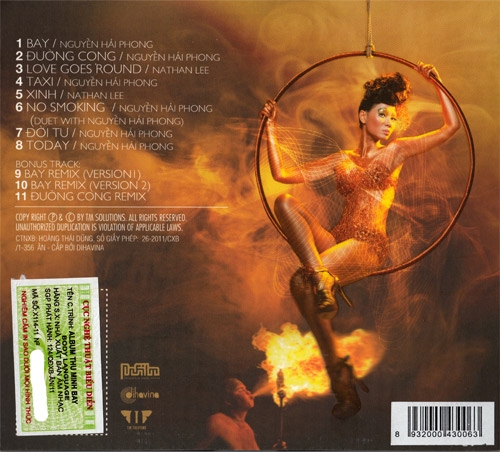The image is likely the back cover of a music CD or album, featuring a central design that includes a woman sitting in a metallic, copper-like hoop swing hanging from a rope. She is dressed in a scanty, copper-colored outfit with very high heels and has her hair up. Her pose shows one leg crossed over the other, and her arms resting on the right and left of the hoop. The background is a smoky, golden-brown, and gray melange that blends with fiery elements, giving an impression of flames behind her. In the top left corner, there is a column of 11 white numbers beside which are white titles, possibly the names of songs, such as “Bay,” “Duong Kong,” and “Love Goes Round." Under the list, there is a white line and then some additional white text, likely indicating bonus tracks. The bottom left of the image features a white-bordered rectangle with a green background and red and white text, oriented sideways, resembling a ticket. Adjacent to it, more text runs vertically down the side. The bottom right corner contains a barcode, solidifying its appearance as a professional cover. The colors in the image include blacks, whites, greens, reds, oranges, yellows, tans, and grays, creating a vibrant yet cohesive visual effect.